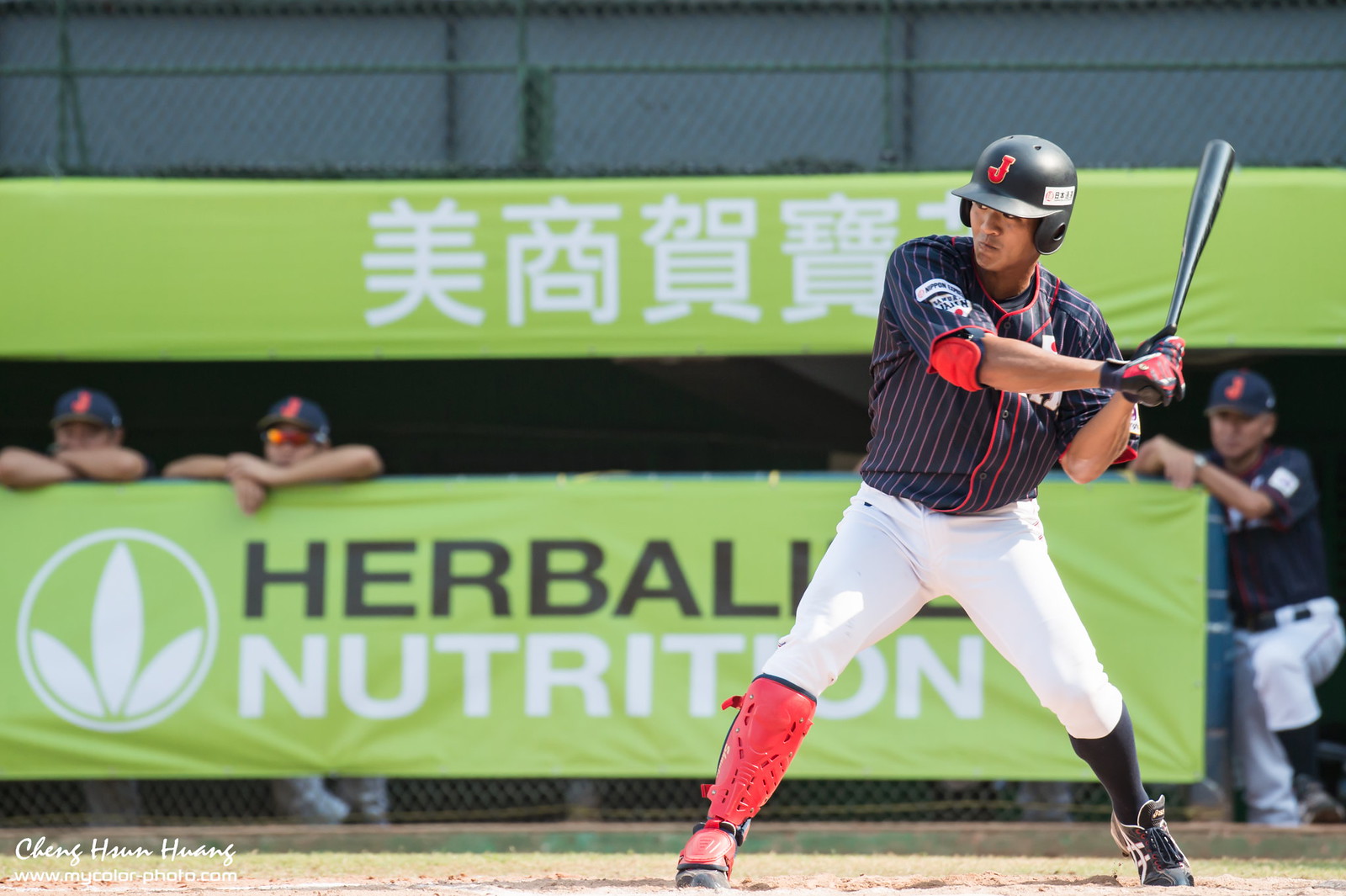This photograph captures a left-handed Japanese baseball player in mid-swing during a game. He dons a black helmet with a red 'J' on it and wears a dark blue jersey adorned with red pinstripes, paired with white pants. His right leg, the leg closest to the pitcher, is protected by an orange shin guard. He swings a black bat, and his left foot sports a black cleat and stocking. Adding to his professional appearance, he has on batting gloves. The backdrop of the image features the bullpen, where his teammates and coach lean against a railing with a light green banner displaying "Herbalife Nutrition." The banner is flanked by Japanese characters above it, indicating the player's likely Japanese heritage. There is also an artist credit at the bottom left, marked "QingHuanHuang www.mycolorphoto.com."